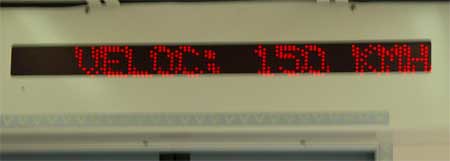This image captures a modern entryway, highlighting a long, rectangular digital screen positioned above the doorway at the bottom of the photograph. The screen prominently displays the text "VELOC 150 km/h," indicating a speed of 150 kilometers per hour. The doorway and surrounding walls are uniformly white, creating a clean and minimalistic aesthetic. Additionally, a long, illuminated white strip runs horizontally in front of the door, further enhancing the sleek, contemporary design of the space.